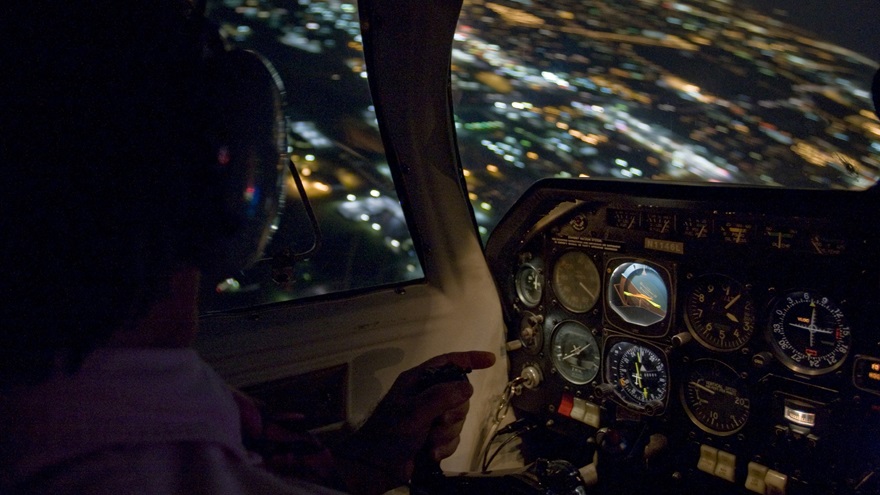The nighttime photograph captures the interior of a cockpit, likely within a helicopter or airplane. The central focus is on a pilot, distinguishable by a helmet and possibly a purple shirt, who is pointing towards an array of gauges and dials on the control panel. The cockpit is illuminated with backlit gauges displaying varied colors such as oranges and blues, corresponding to aircraft instruments including altitude gauges, speed gauges, RPM indicators, and angle-of-attack meters. Beneath these gauges, switches and buttons are visible, and notably, a key is situated in the ignition.

Through the cockpit glass, the image reveals a blurry night-time cityscape, illuminated by the distant lights of businesses, houses, and street lamps on the ground below. The angle of the shot suggests the aircraft is slightly banked, further blurring the city view. The overall darkness of the image emphasizes the lit instruments and the illuminated ground below, creating a stark contrast in the photo. While the pilot's head is not entirely visible, the orientation and the headset suggest active engagement in flying the aircraft. The detailed elements within the cockpit—along with the night-time setting—create a vivid and dynamic portrayal of the flight experience.